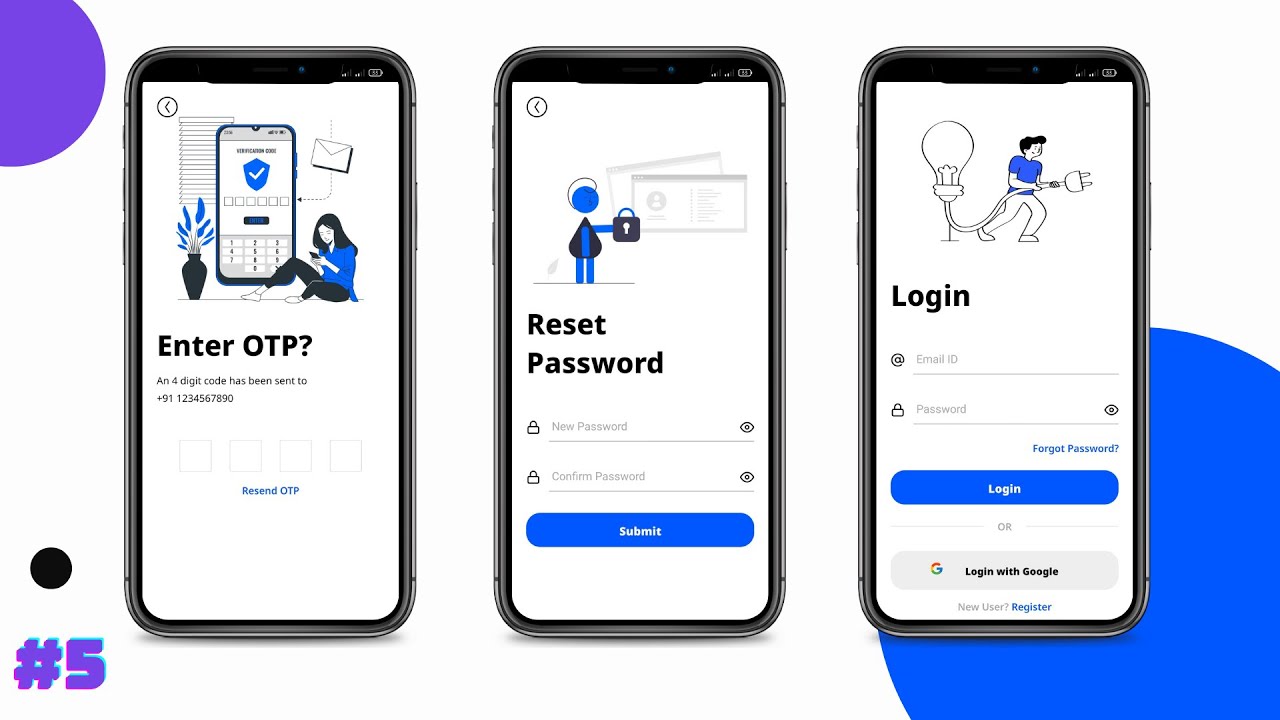**Descriptive Caption:**

"This image is a screenshot of an instructional page from a mobile application, showcasing three distinct yet stylistically similar phone screens. Each screen presents a different step in a user authentication process.

1. The leftmost screen prompts the user to 'Enter OTP?' with the message: 'A four-digit code has been sent to [phone number].' It includes an option to resend the OTP.
  
2. The middle screen is dedicated to resetting the password. It features two input fields: one for entering a new password and another for confirming it. A 'Submit' button is also present.

3. The rightmost screen is the login interface, containing fields for 'Email ID' and 'Password,' along with options for 'Forgot Your Password?' and a 'Login' button. Additionally, there's an 'Or Login with Google' button for alternate authentication.

Each screen is adorned with cute, minimalist cartoon sketches in a color scheme of black, blue, and white, maintaining a cohesive and user-friendly aesthetic throughout the app interface."